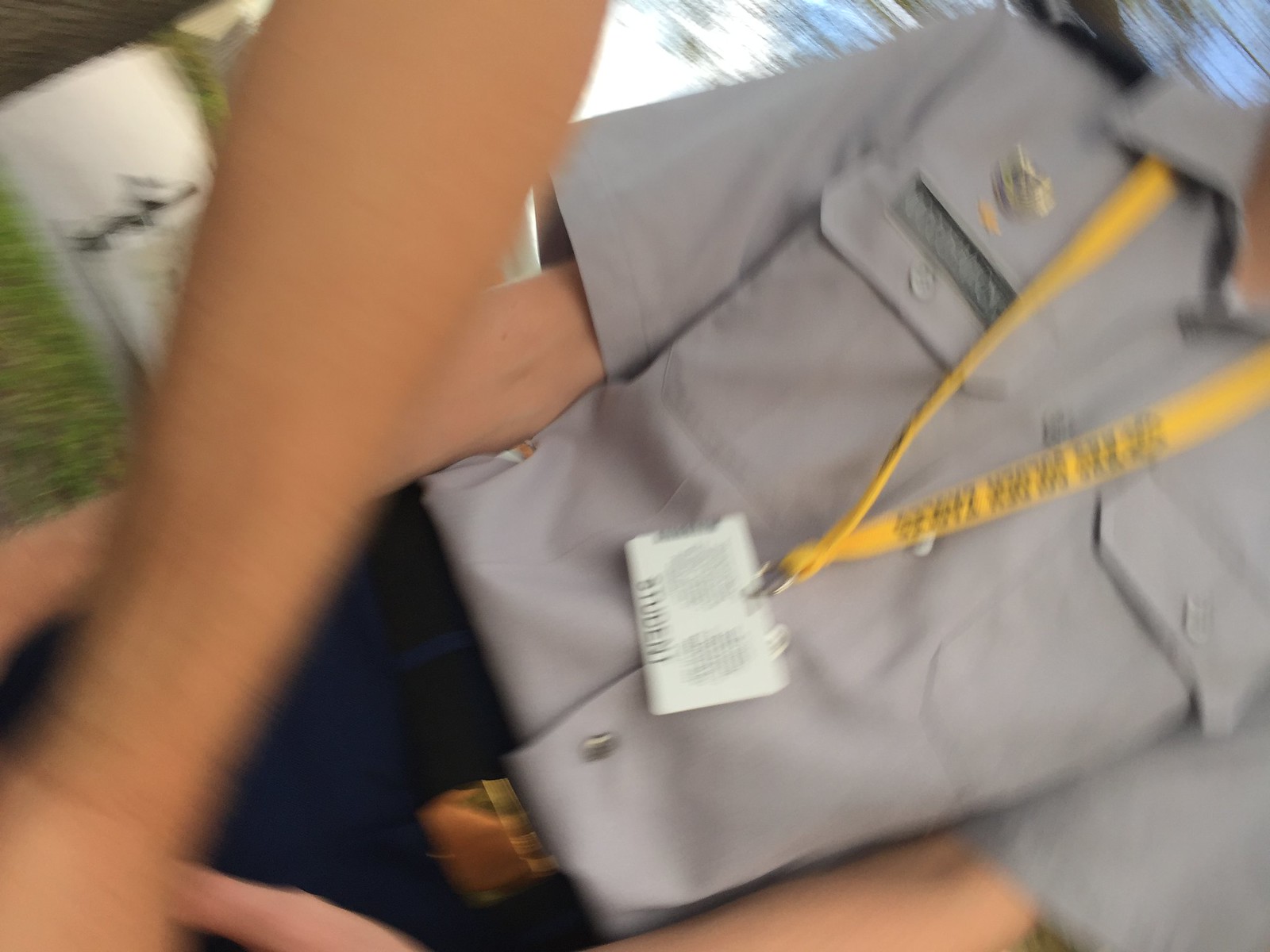A color photograph, oriented sideways in a landscape format, showcases a young man in a military-style uniform. The image captures him from the neck downward, highlighting the details of his attire. He wears a yellow lanyard with an attached badge around his neck. On the right breast pocket of his uniform, there is a name patch accompanied by a small metal pin above it. The man holds his arms straight down in front of him, and he appears to be holding hands with someone whose arm extends over his body and out of the frame toward the bottom left corner. This second person's torso is visible from the side, clad in the same uniform, extending down to mid-thigh, but their identity remains obscured.